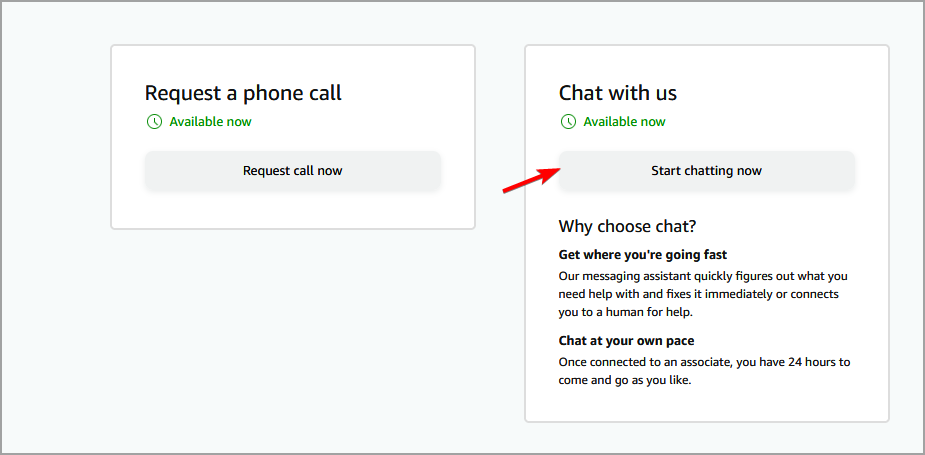This image depicts a clean, white screen interface commonly seen on websites. Two interactive pop-up boxes are prominently displayed. 

On the left, a box offers an option to "Request a Phone Call." It emphasizes availability with the message, "Available Now," and includes a clickable button labeled "Request Call Now."

On the right, a contrasting pop-up provides a chat option and is labeled "Chat with Us." It, too, highlights immediate availability with the phrase, "Available Now," and features a button that invites users to "Start Chatting Now."

The chat box elaborates on the benefits of choosing the chat feature: 

1. **Get Where You're Going Fast**: The messaging assistant quickly identifies the user's needs, offers immediate solutions, or connects the user to a human representative if necessary.
2. **Chat at Your Own Pace**: Once connected with an associate, users have the flexibility to continue the conversation for up to 24 hours at their convenience.